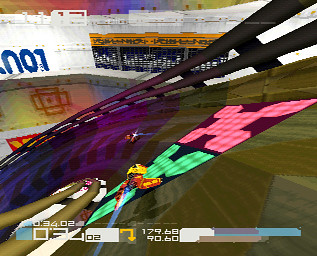In this vibrant and slightly blurry screenshot from a futuristic racing video game, reminiscent of Wipeout, we see sleek, triangular-bodied spaceships racing along a track. Dominating the center of the image is a bold, red and yellow spacecraft with jet boosters, zooming over a green X symbol. Adjacent to it is a pink X symbol, hinting at various in-game features such as power-ups or boosts. In the distance, another spaceship follows a blue arrowed path, set against a somewhat ambiguous white background with possibly non-English text. The bottom portion of the screen displays numerical stats in white text: 34.02, 179.68, and 90.60, accompanied by a multicolored health meter. The overall scene is awash with bright, dynamic colors and intricate geometric patterns, capturing the essence of high-speed, futuristic racing.